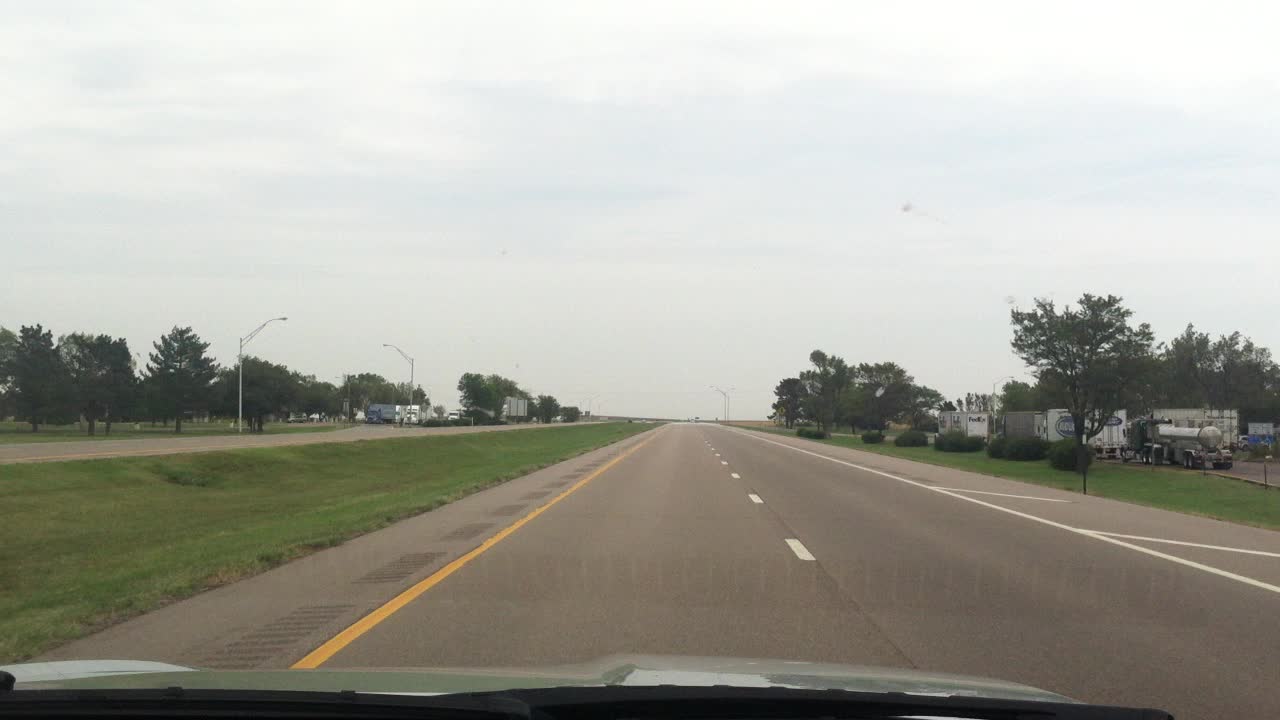This daytime photograph, taken from within a green-colored vehicle, presents a clear, detailed view of a four-lane highway. The image is captured from the left-hand inside lane of the highway, with the vehicle's hood visible at the bottom of the photo. The highway is divided by a grass median separating two lanes in each direction. To the left of the car, the grass median is prominent, leading to the lanes heading in the opposite direction.

On both sides of the highway, there are areas designated for truck parking, populated with several semi-trucks. Trees line the horizon on both the left and the right, with the road extending straight into the distance until it meets the sky. The edges of the road are clearly marked by a solid white line on the right, a dashed white line in the center, and there are faint traces of streetlights and a building visible in the distance.

The sky, occupying the upper half of the photograph, is a mix of light white and streaks of blue, giving the appearance of an overcast or partly cloudy day. The photograph is brightly lit and in sharp focus, with no other vehicles visible on the road. There are no inscriptions or text within the image. Overall, this image captures a serene and expansive view of the highway stretching towards the horizon.